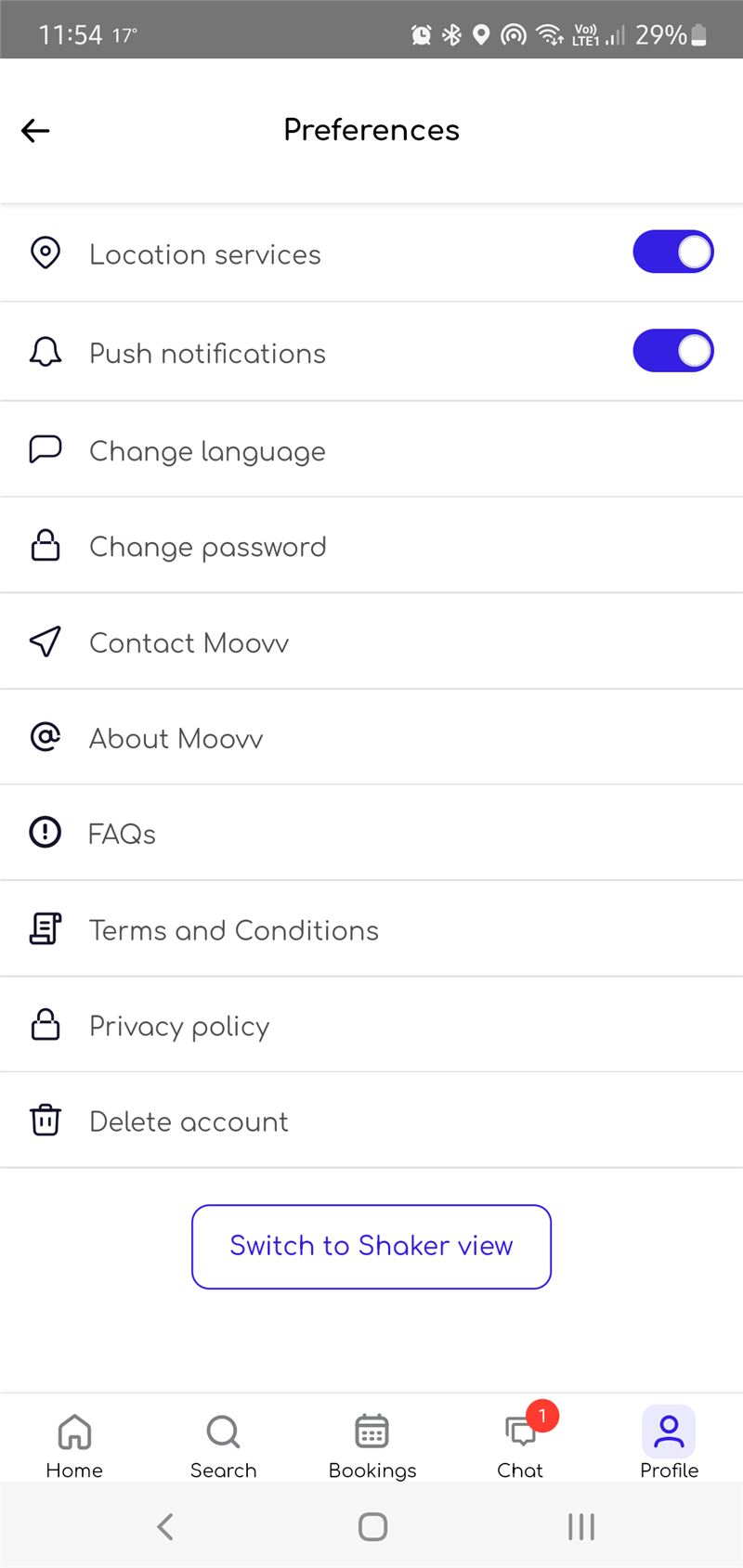The image displays a smartphone's 'Preferences' page, captured from the device's screen. The left side of the screen is populated with a vertical row of icons, each representing different settings. At the top of the screen, there is an icon of a pin, labeled 'Location Services', accompanied by a slider on the far right that is toggled on. This is depicted by a royal blue background behind the white circular slider, indicating its active status.

Below this, a bell icon is labeled 'Push Notifications', with a similar slider on the right currently toggled off. Next, a speech bubble icon represents 'Change Language', though it lacks an associated slider. This is followed by a lock icon labeled 'Change Password'. Additional sections listed below include 'Contact Us', 'About Us', 'FAQs', 'Terms and Conditions', 'Privacy Policy', and 'Delete Account'. At the very bottom of the page, there is a button labeled 'Switch to Shaker View.' The interface is clean and navigable, displaying essential user preferences in a structured manner.